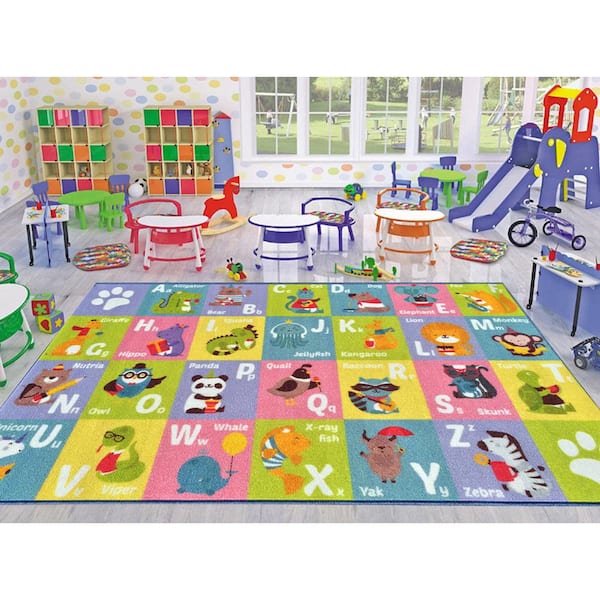The image depicts an inviting and colorful preschool play area that's bursting with various elements. Dominating the center of the room is a large, vibrant alphabet rug, where each letter from A to Z is paired with a corresponding animal illustration, such as an owl for "O" and a zebra for "Z". The rug is made up of multicolored squares and serves as a focal point in the room. 

Towards the back, there is a collection of child-sized furniture, including a table surrounded by chairs in a rainbow of colors: blue, green, red, and orange. Adjacent to the seating area is a small slide designed to look like an elephant; it features a red top with small windows and a yellow roof that adds a whimsical touch.

On one side of the room, five large windows flood the space with natural light and offer a view of an outdoor playground where children are seen playing on swings and other equipment. To the left of the play area, two multicolored cabinets in shades of green, orange, and blue provide storage space, likely for toys and supplies.

Additional details include white wallpaper adorned with colorful polka dots, adding to the playful atmosphere. There are also various other play items scattered around, such as a small xylophone table, a tricycle, a rocking horse, and a couple of green cables positioned to the left and right. The scene exudes a lively and engaging environment designed for young children to explore and learn.